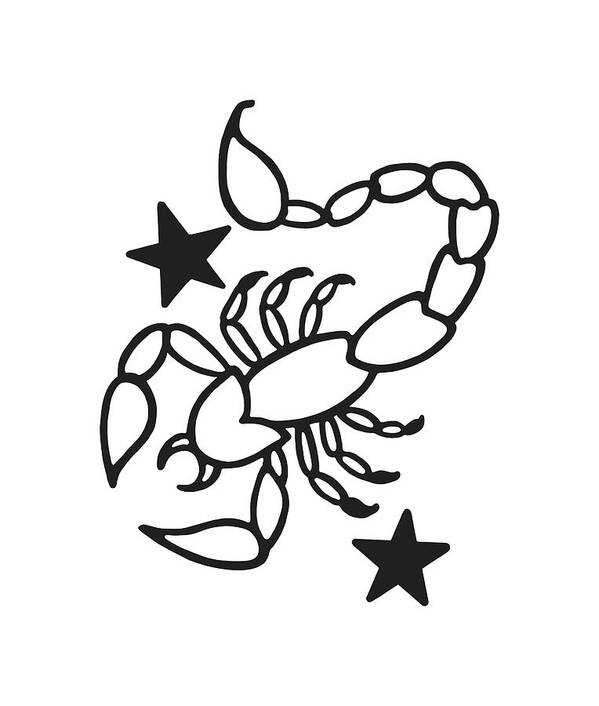This is a black and white illustration of a scorpion, often associated with the Scorpio zodiac sign. The scorpion is outlined in bold black brush lines, creating a striking, simplified depiction reminiscent of a tattoo design or a coloring book illustration. It features six legs, two pincers at the front, and an additional pair of pinchers emanating from its mouth. The creature is oriented diagonally, facing the bottom left, while its tail curls upwards to the right and ends in a sharp stinger pointing towards the top of the image. The backdrop is a stark white, and the scene is framed by two solid black, five-pointed stars—one positioned above the scorpion to its upper left, and the other below it to its bottom right.